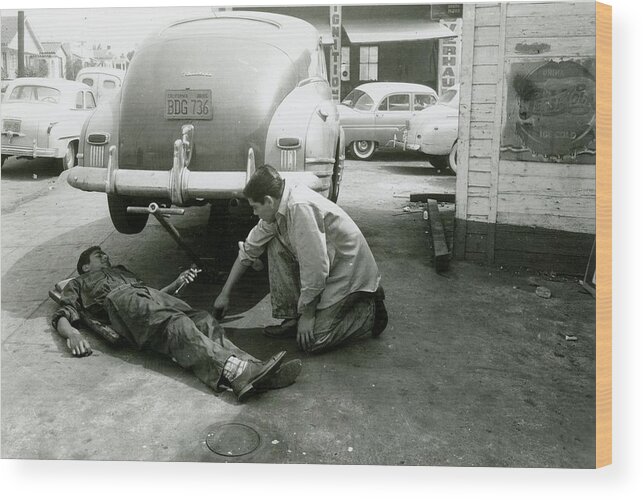This illuminating black-and-white photograph, likely from the 1940s or 1950s, captures the bustling activity of a mechanic shop during the day. A classic car, jacked up high, dominates the foreground, casting a distinct shadow that hints at the time of day. The car, with its rounded back and high window, bears the license plate BDG 736. To the right, a wooden building displays a fainted Pepsi-Cola advertisement, emphasizing the bygone era. The building features a lighter upper exterior and a darkly painted lower border. In the center of the scene, a mechanic clad in overalls lies on a rolling board beneath the jacked-up car, a wrench firmly in his grasp. His light-skinned colleague, dressed in a long, light-colored shirt with rolled-up sleeves and bent on one knee, leans down to converse with him. The background reveals more antique cars parked, reinforcing the setting as a traditional auto repair shop.